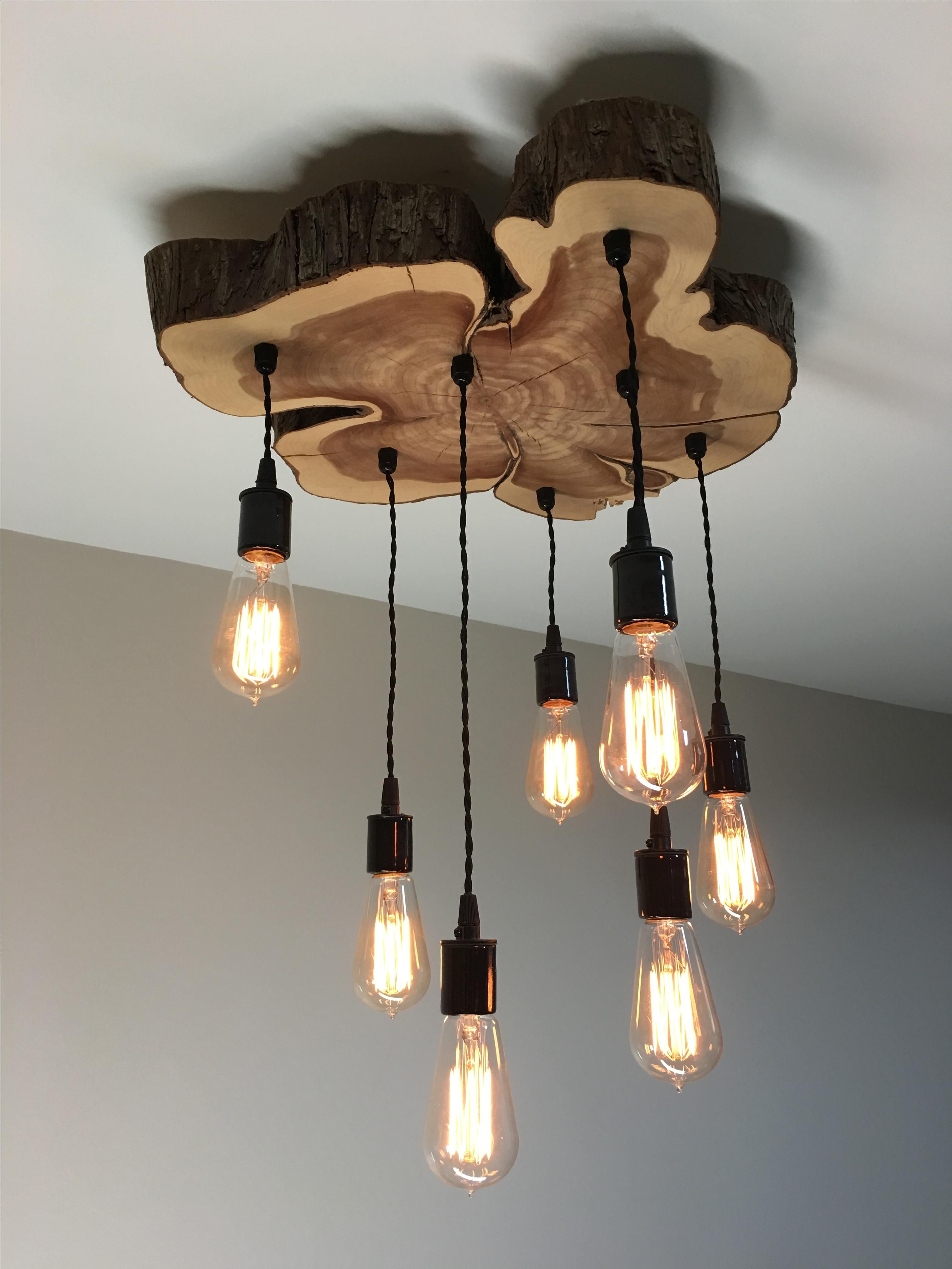The image depicts a rustic, homemade chandelier affixed to a white ceiling. The chandelier's base is an asymmetrical, roughly cut slab of tree trunk, approximately four to five inches thick. This slab features visible tree rings and retains its natural bark, presenting a blend of light and dark browns that emphasize its origin. Hanging from this wooden base, seven vintage-style light bulbs are suspended at varying heights by black wires, contributing to an old-fashioned aesthetic. The bulbs emit a light yellowish to amber glow, enhancing the chandelier's warm, nostalgic feel. The backdrop includes a light to medium gray wall, further highlighting the chandelier's distinct features.